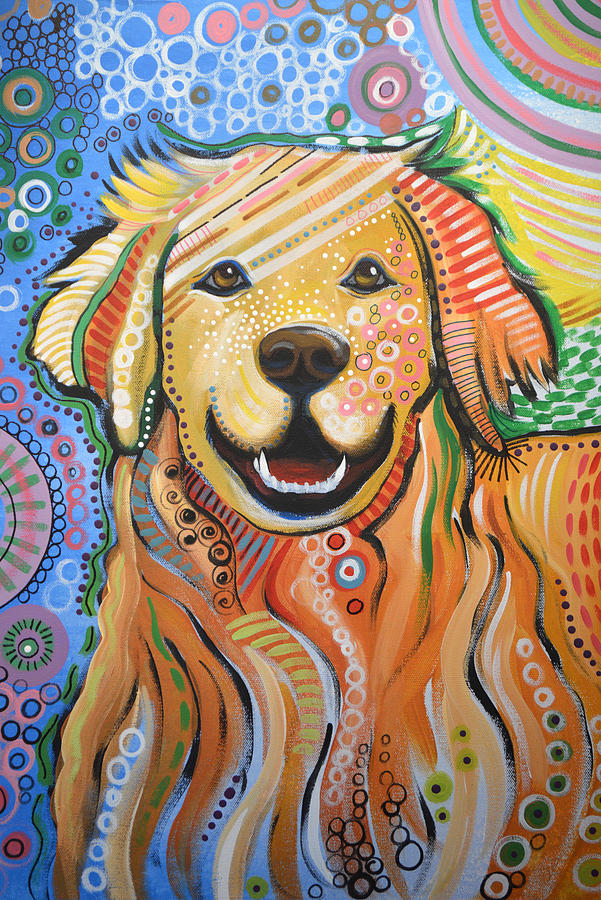This detailed, vibrant oil painting features a smiling Golden Retriever prominently in the center. The portrait is vertically oriented, longer in height than width. The dog's face is beautifully shaded with a mix of colors, primarily showcasing a tan base adorned with an array of white freckles. Intricate designs with pink and white circles decorate the area beneath its expressive brown eyes, which are highlighted with subtle blue liner. The retriever's ears are painted in an eclectic mix of horizontal and vertical lines, featuring hues like red, pink, blue, green, yellow, and white.

The dog's body continues this colorful theme, predominantly covered in long strands of orange fur, interspersed with light blue, white, and green strands. The painting's background is a rich blue, teeming with dynamic patterns that add a sense of depth and whimsy. Various sized circles, including green, white, and black, populate the space behind the dog, creating a light-hearted, almost "trippy" atmosphere. The combination of these playful colors and intricate designs makes this Golden Retriever painting a striking centerpiece.